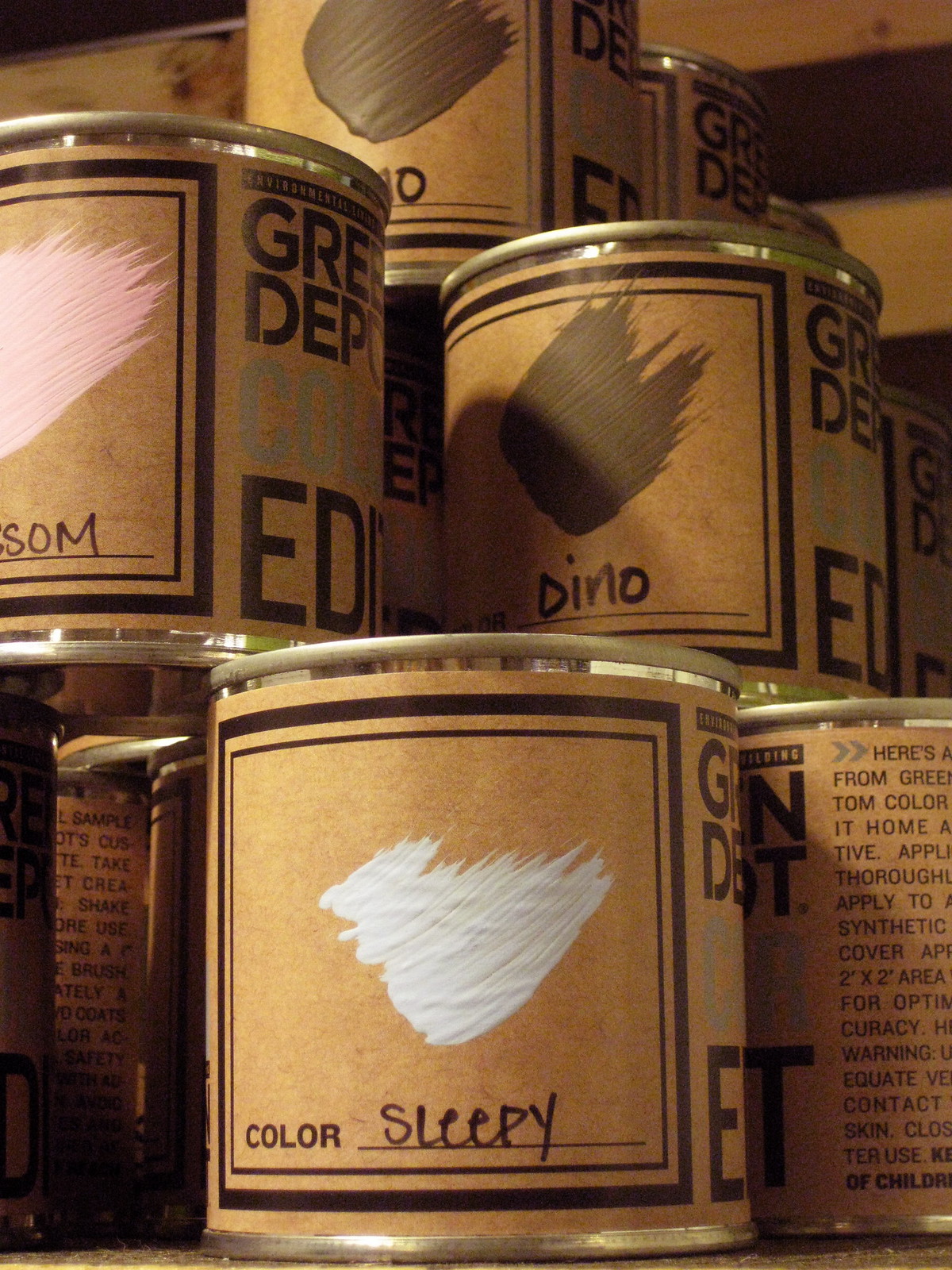This sepia-toned image captures an arrangement of small, silver paint cans stacked atop one another in a setting that resembles a warehouse. Each can is adorned with a cardboard-like label, designed with a tan or brown hue and a square border specifically for showcasing the paint color. Prominent among the cans is one at the bottom, labeled "Sleepy," which features a white paint swatch. Another can displays a pink swatch, possibly named "Blossom," and yet another on top has a black paint swatch, with a name that looks like "Darlow" or "Dino." Each can has a silver top and a label space where the color's name is written beneath the swatch. There is text in the background, partially obscured by the stack of cans, adding to the industrial and cluttered atmosphere of the scene.